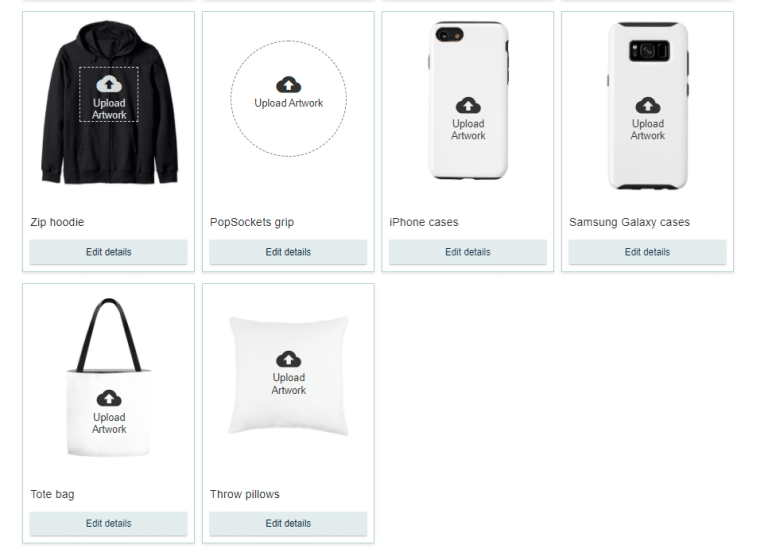The image displays a series of six products available for customization on an e-commerce website. Each product slot contains an illustrative placeholder indicating where a user can upload their own artwork:

1. **Zip Hoodie**: Depicted in black and white, the zippered hoodie features a square placeholder with an upload icon. Beneath the icon, there is a label stating "Upload Artwork" with a button labeled "Edit Details" at the bottom.

2. **Pop Sockets Grip**: To the right of the zip hoodie is a circular placeholder intended for a custom pop socket. It includes an upload icon within a dotted circle. Below this, the text reads "Upload Artwork," and there is a button for "Edit Details."

3. **iPhone Case**: The next item is an iPhone case shown in white with a centered upload icon on its back. The accompanying text "Upload Artwork" appears below the icon, along with a button labeled "Edit Details."

4. **Samsung Galaxy Case**: Similar to the iPhone case, this item is displayed with a cloud and arrow upload icon. The text reads "Upload Artwork," and there is a button named "Edit Details" beneath it.

5. **Tote Bag**: The tote bag is illustrated in a black-and-white design with an upload icon placed centrally. Below the icon is the instruction "Upload Artwork," accompanied by a button for "Edit Details."

6. **Throw Pillow**: The final product is a throw pillow, featuring a cloud-shaped upload icon. Underneath, the text reads "Upload Artwork," with a corresponding button labeled "Edit Details."

Each product is shown without any pre-existing designs, inviting customers to personalize them by uploading their unique artwork.